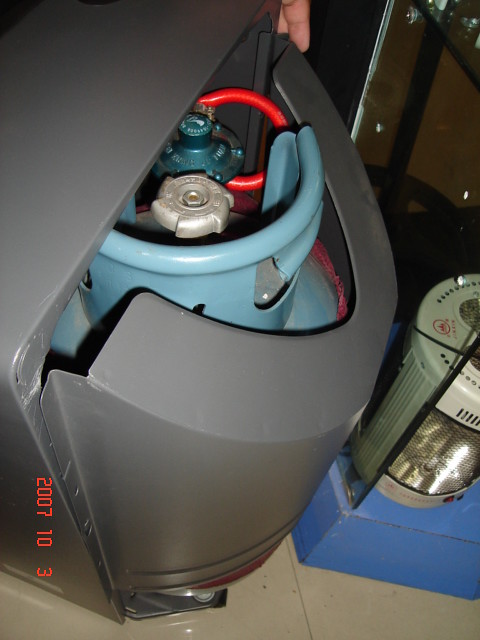The photograph features a hot water heater encased in grey metal, looking relatively new without any visible rust. The image is taken from above, providing a clear view of two knobs at the top of the heater—one silver and one blue. An orange metal pipe descends from the unit. To the right of the heater, there is a blue metal square box supporting a fluorescent style lantern with a green casing. The floor beneath is covered in tan-colored linoleum with lines. At the top center of the photograph, a person's hand is visible, and an orange stamp at the bottom left corner indicates the date 2007-10-3. The overall setting suggests a utility space possibly in a basement or pantry.